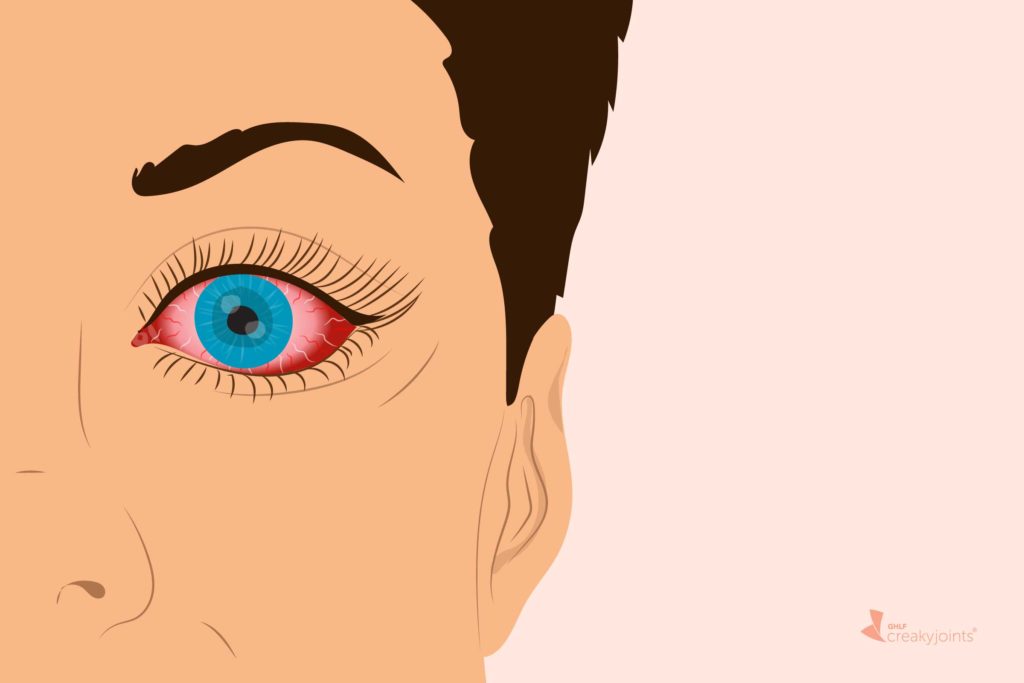This image depicts a detailed graphic of a partial human face set against a light pink background. The focus is primarily on the left side of the face, which prominently features an eye with a vibrant blue iris and red veins, providing a striking contrast. The eye is framed by dark brown eyelashes and a matching eyebrow above. The facial skin is depicted in a light brown hue, and only part of the face, including the eye, a portion of the nose, and the ear, is visible. The hair, which is short and dark brown, along with the ear, adds to the intricate details of the graphic. Notably, the bottom right corner of the image displays the text "CREAKY JOINTS" alongside a dark pink logo.